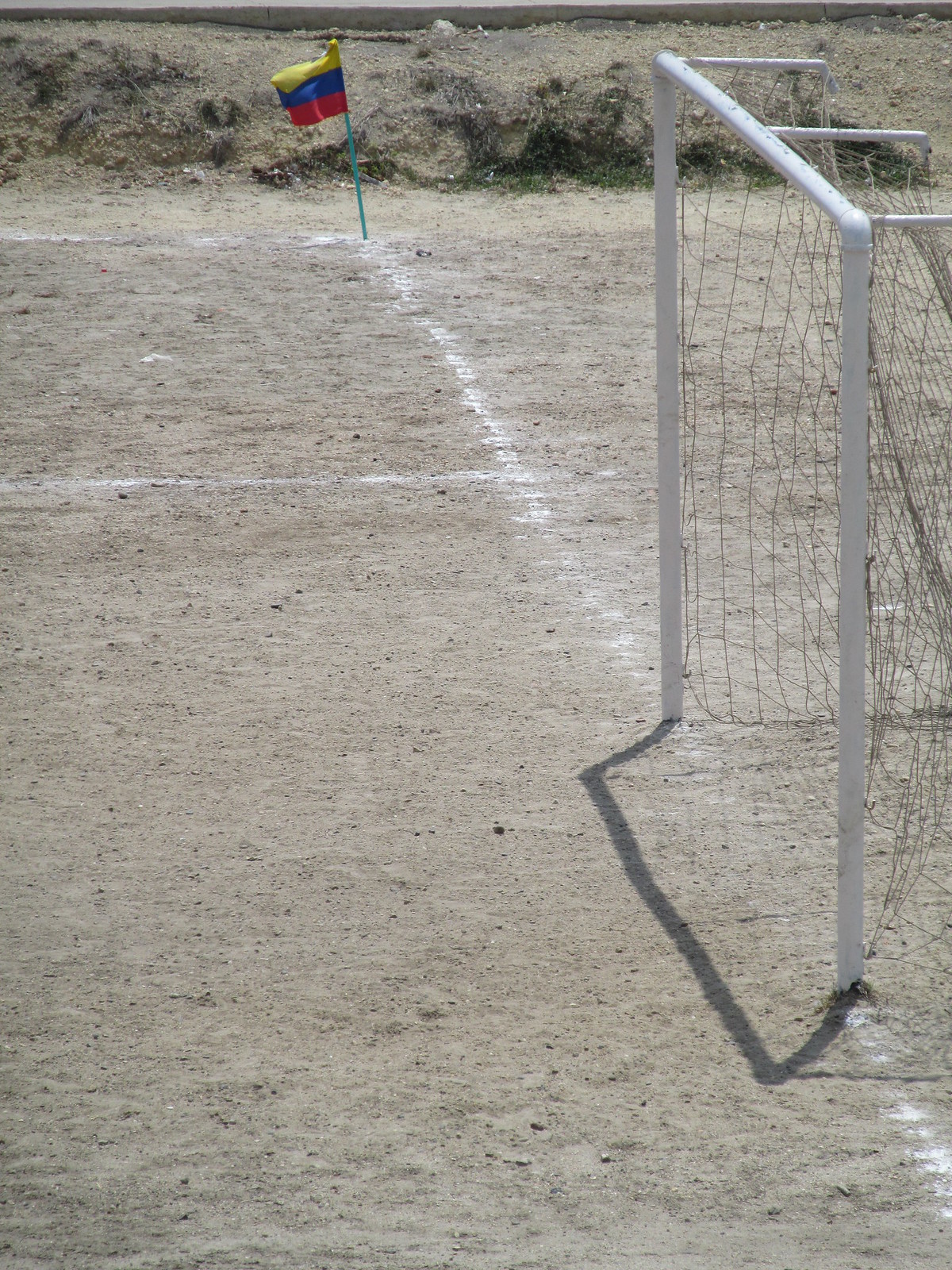This is a full-color photograph taken outdoors during a bright day, showcasing a run-down recreational field. Dominating the foreground is a small soccer or field hockey goal, constructed from a white PVC-type frame and fitted with a dark net. The goalposts appear somewhat makeshift and are firmly staked into the sandy ground. Surrounding the goal are several white chalk lines marking the field boundaries, extending vertically under the goal and continuing across the dirt-covered terrain.

To the left of the goal, staked into the soil, is a small flag with distinct horizontal stripes: yellow on top, blue in the middle, and red on the bottom, attached to a green pole. Another voice mentioned the presence of a yellow, blue, and green flag, but with a pole that appears blue.

In the background, the field transitions to patches of dead grass and small mounds of dirt, coupled with sporadic patches of scrub brush. The scene is marred by litter, reflecting a neglected environment. Notably, there are no people present, emphasizing the isolation and abandonment of this field.